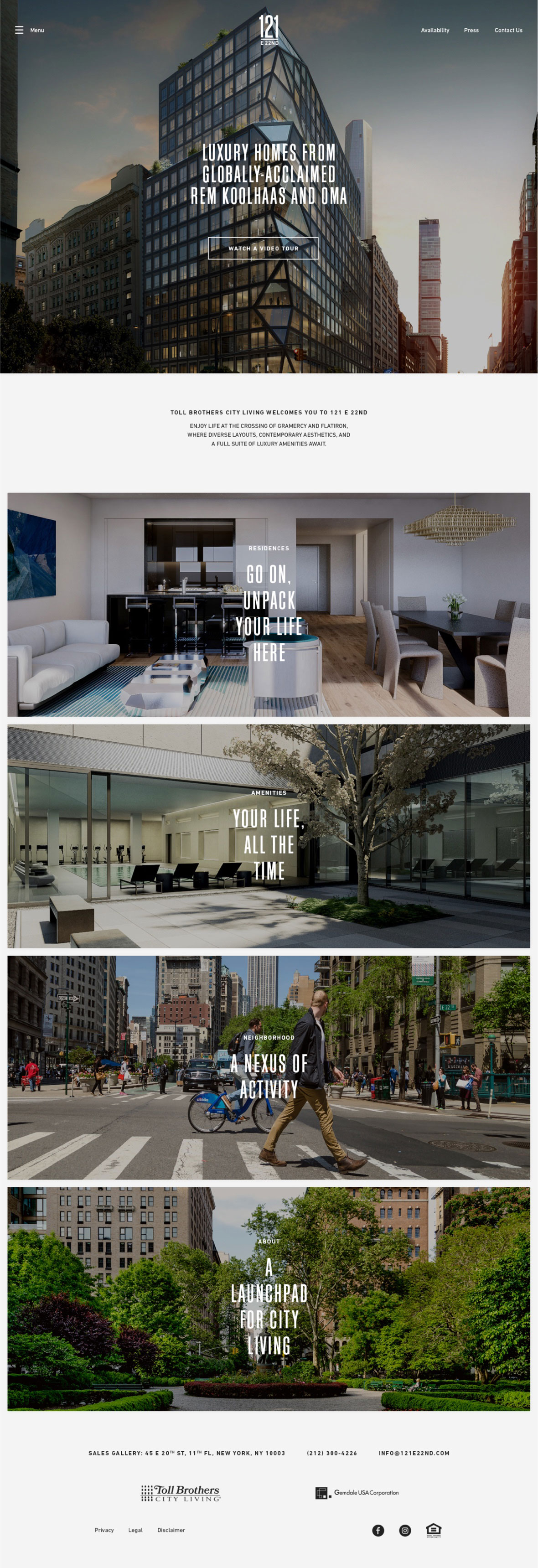Discover Toll Brothers City Living's newest development at 121st East 22nd. Introducing a prime locale at the heart of Gramercy and Flatiron, where urban sophistication meets modern convenience.

The advertisement's top image showcases the sleek, glass facade of the building, its transparent design framed with black outlines. Warm yellow lights illuminate the interiors, creating an inviting atmosphere. The website navigation is clearly displayed: "Menu" on the left, "Availability," "Press," and "Contact Us" on the right, set against a pristine white background.

Central to the ad is the welcoming message: "Toll Brothers City Living welcomes you to 121st East 22nd. Enjoy life at the Corset of Gramercy in Flatiron, where diverse layouts, contemporary aesthetics, and a full suite of luxury amenities await."

The second image provides a glimpse into a stylish apartment, featuring a white couch, complemented by a brown table on the right and a gold chandelier above—a true epitome of modern interior design. The text in white invites you to, "Residences Go On. Unpack your life here."

Next, the amenities section is highlighted with an image of a state-of-the-art gym. It includes treadmills and a luxurious Olympic-sized pool lined with comfortable pool chairs. The accompanying text reads, "Amenities: your life all the time."

Following this is a bustling street scene of New York City, capturing the essence of local life with people walking about. The caption, "Neighborhood: a nexus of activity," encapsulates the vibrant energy surrounding the development.

Finally, the bottom image portrays the neighborhood's skyline, dotted with gray buildings amidst lush green and red foliage. The concluding message, "About: a launchpad for city living as well," reinforces the prime, nature-infused urban lifestyle offered at 121st East 22nd.